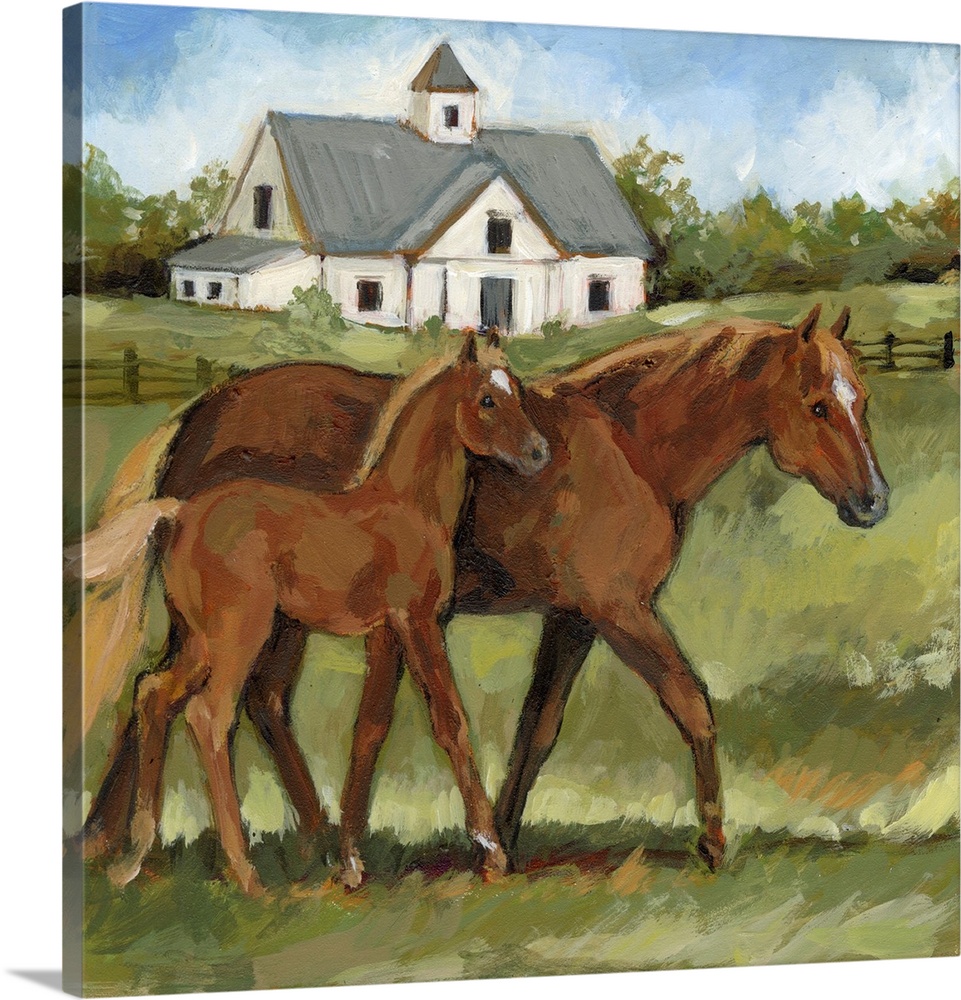The painting depicts a tranquil pastoral scene with a brown, wooden fence surrounding a lush, green pasture. In the foreground, there are two brown horses—an adult mare and a foal. Both horses have distinctive blonde manes and tails, along with a white diamond-shaped marking between their eyes. The foal stands close to the mare, suggesting a nurturing bond. In the background, beyond the fence, stands a large white house featuring a gray, triangular roof and a small lookout at the top. The house is set against a backdrop of trees and bushes, under a bright blue sky filled with fluffy white clouds. The painting is rendered in long, sweeping brush strokes that give it a textured, almost impressionistic feel.